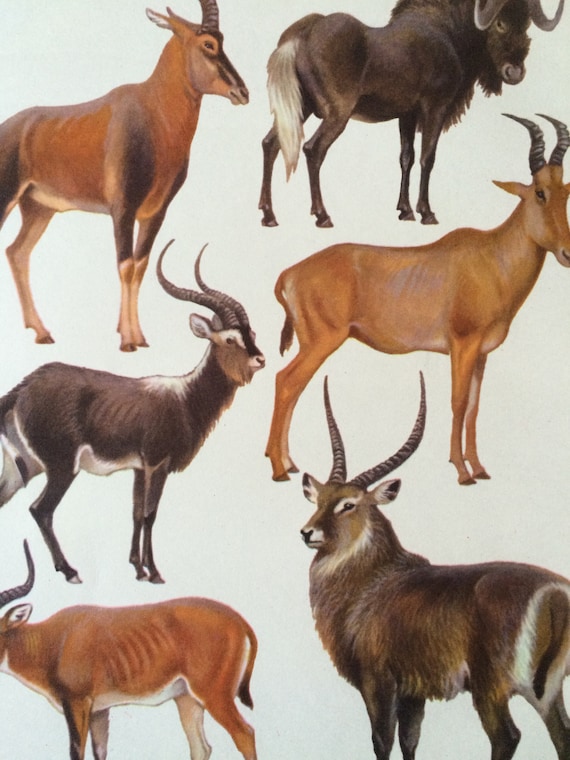The image features a detailed drawing of six large horned animals, which appear to be various species of goats, ibex, elk, and buffalo. They are arranged in two vertical columns of three animals each. On the left side, the animals alternate colors from light brown, to dark brown, to light brown again. The right column alternates from dark brown, to light brown, to dark brown. All of the animals are standing on four legs and have distinctive horns. The dark brown animals in the upper right, middle left, and bottom right have antlers, with the upper right one displaying curved antlers that descend and then ascend like those of a buffalo. The middle and bottom right dark animals have upward-curving antlers more reminiscent of a goat. The light brown animals, on the other hand, have uniform brown coats, except for the lower left one which has a white undercoat. The background is a plain, very light green with a grayish tint, emphasizing the intricacies of each drawn animal.